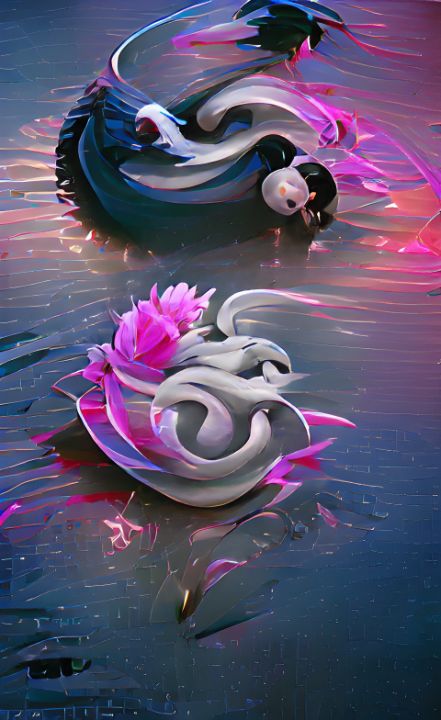This highly stylized abstract painting features a dynamic color palette dominated by dark blues, grays, blacks, vibrant pinks, purples, and light whites. The image portrays elements suggesting swans or birds on a body of water, blending seamlessly with their surroundings. One swan, painted dark, contrasts with another swan or bird that is white and adorned with pinkish-purple flower-like shapes. The background is a fusion of soft, horizontal lines that evoke a sense of fluidity and liquid motion, with colors subtly melting into each other. The abstract nature of the image leaves it open to interpretation, evoking a futuristic and visually captivating scene that combines organic elements like flowers or petals floating on a liquid surface with an enigmatic, dreamlike quality.